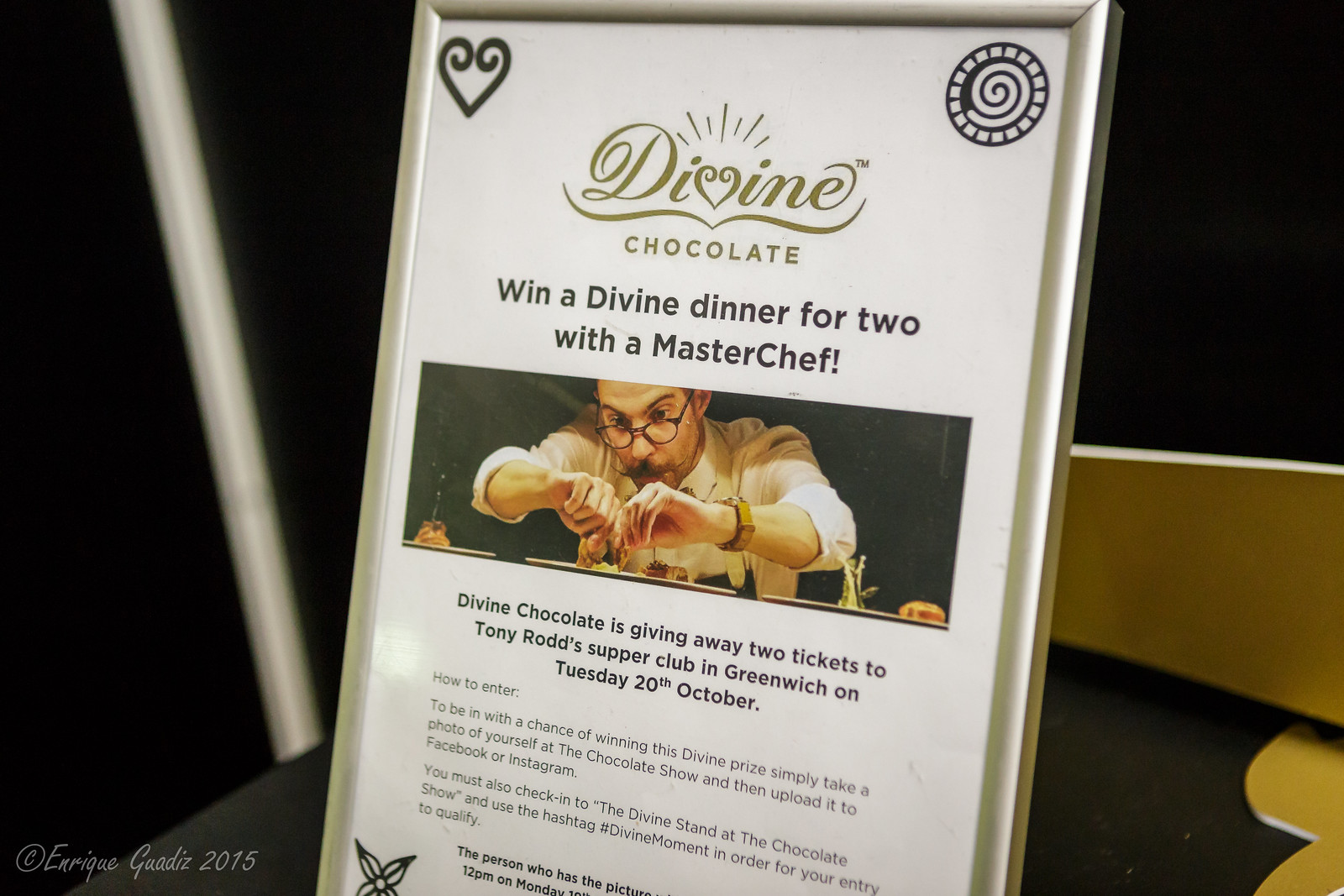In a dimly lit room, a sophisticated advertisement for Divine Chocolate stands out with its elegant presentation. Housed in a gleaming silver frame, the display features an intricate design where the letter V in "Divine" is shaped as a heart. Below, written in luxurious gold letters, is the tagline "Win a divine dinner for two with a master chef." A narrow, rectangular photograph within the frame showcases a gentleman wearing a chef's uniform and dark glasses, presumably the master chef in question, skillfully preparing a meal. Further down, the text announces that Divine Chocolate is offering two tickets to Tony Rod's Supper Club, an exclusive event in Greenwich on Tuesday, October 20th. The advert is set against a background featuring a grayish pole to the left and a golden railing to the right. Additional details, written in smaller print, hint at further information about this opulent contest.